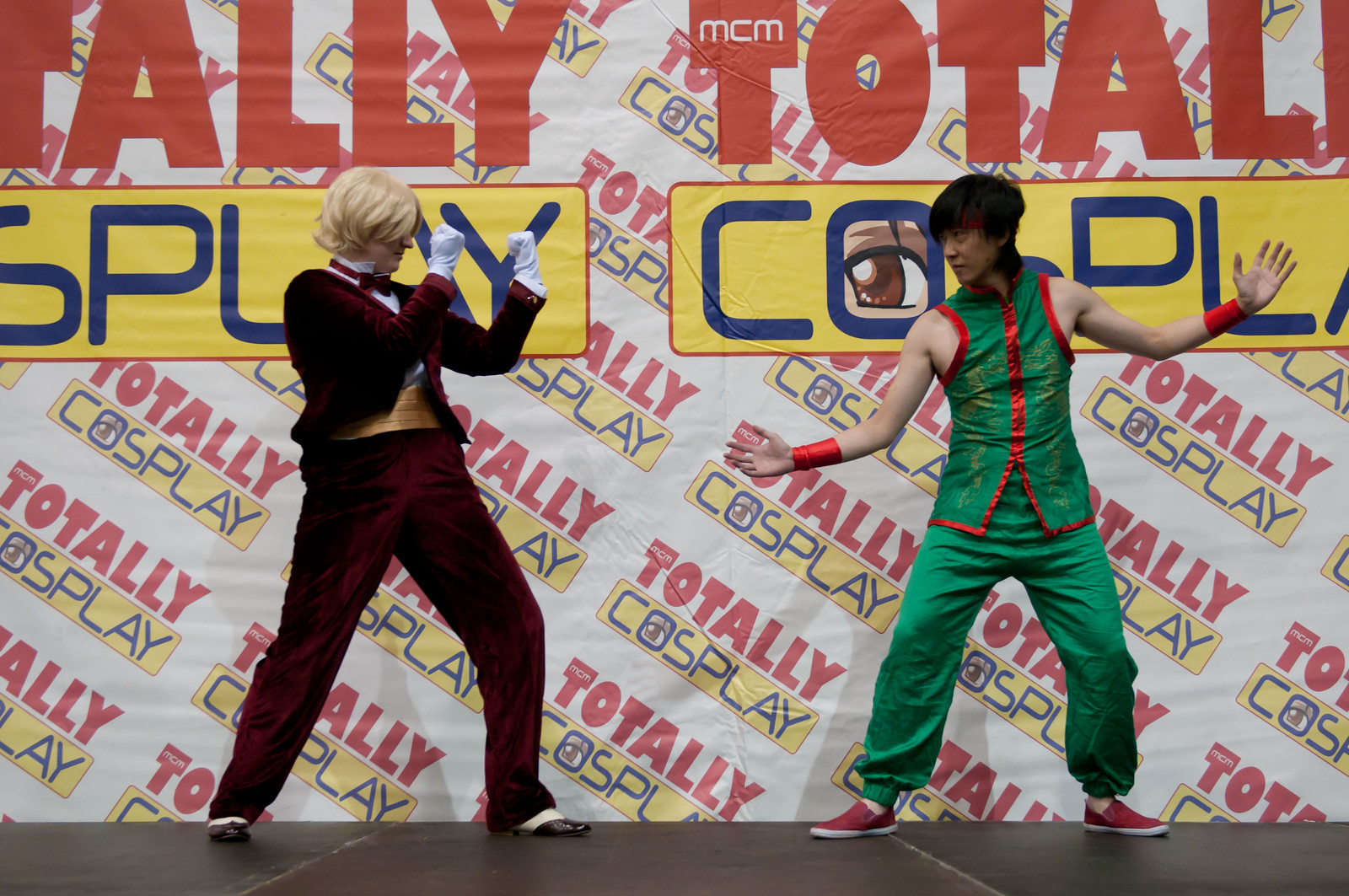This image captures a dynamic scene from a Totally Cosplay convention. On stage, two individuals, one Asian and one white, are depicted in a mock combat pose. The white individual, on the left, sports a blonde, short wig and is dressed in a striking maroon velvet suit adorned with a black bow tie and white gloves. The shirt beneath his open jacket reveals only his chest. The Asian individual on the right has black hair and is clad in a martial arts-inspired green outfit with a red trim, matching pants, and red shoes, completed with red armbands around his wrists. Both are posed as if ready to engage in a fight. The backdrop features the words "TOTALLY COSPLAY" repetitively displayed in red, yellow, and blue lettering against a white background, along with a major sign that reads “Tally Totals Fly Cosplay” above it. The stage is dark brown or black, adding a dramatic contrast to the vividly dressed cosplayers.